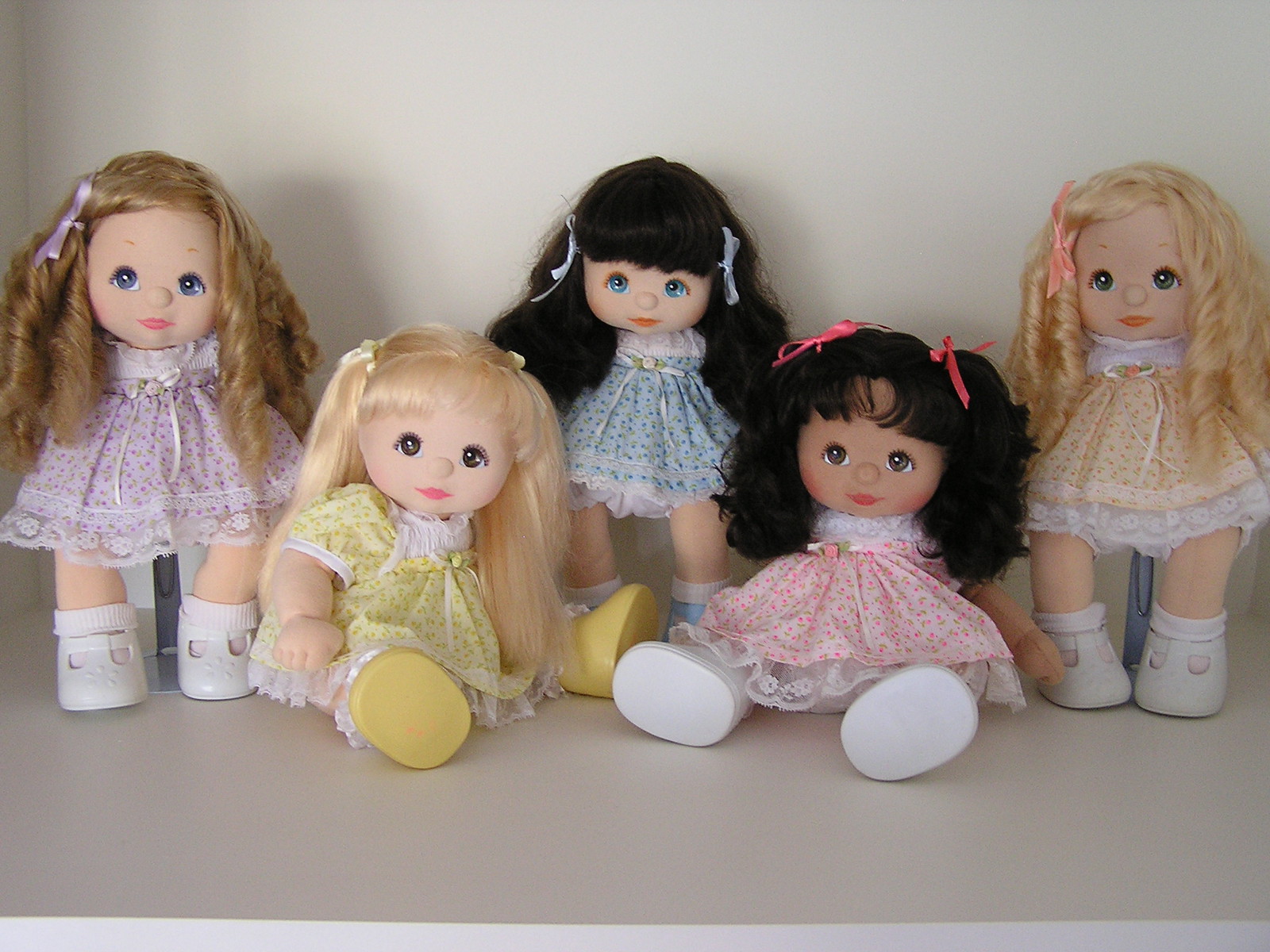The image features a group of five diverse cloth dolls arranged from left to right on a light gray surface, possibly a shelf, against a light gray wall. The first doll on the left stands with long, curly brown hair, adorned in a white dress with pink designs and wearing white shoes. Next to her, a sitting doll with long, straight blonde hair sports a yellow and white dress, revealing yellow shoes that peek out. Behind her, partially obscured, another doll stands with long black hair tied with ribbons, wearing a white and blue dress and showing just a hint of her socks. The seated doll to her right has shoulder-length, curly black hair, a pink and white dress, and visible white shoe bottoms. Finally, on the far right stands a doll with curly, long blonde hair, featuring a ribbon on her left side and wearing a gold-tinted white dress with white shoes. The entire ensemble is set against a neutral, off-white to tan-beige background.